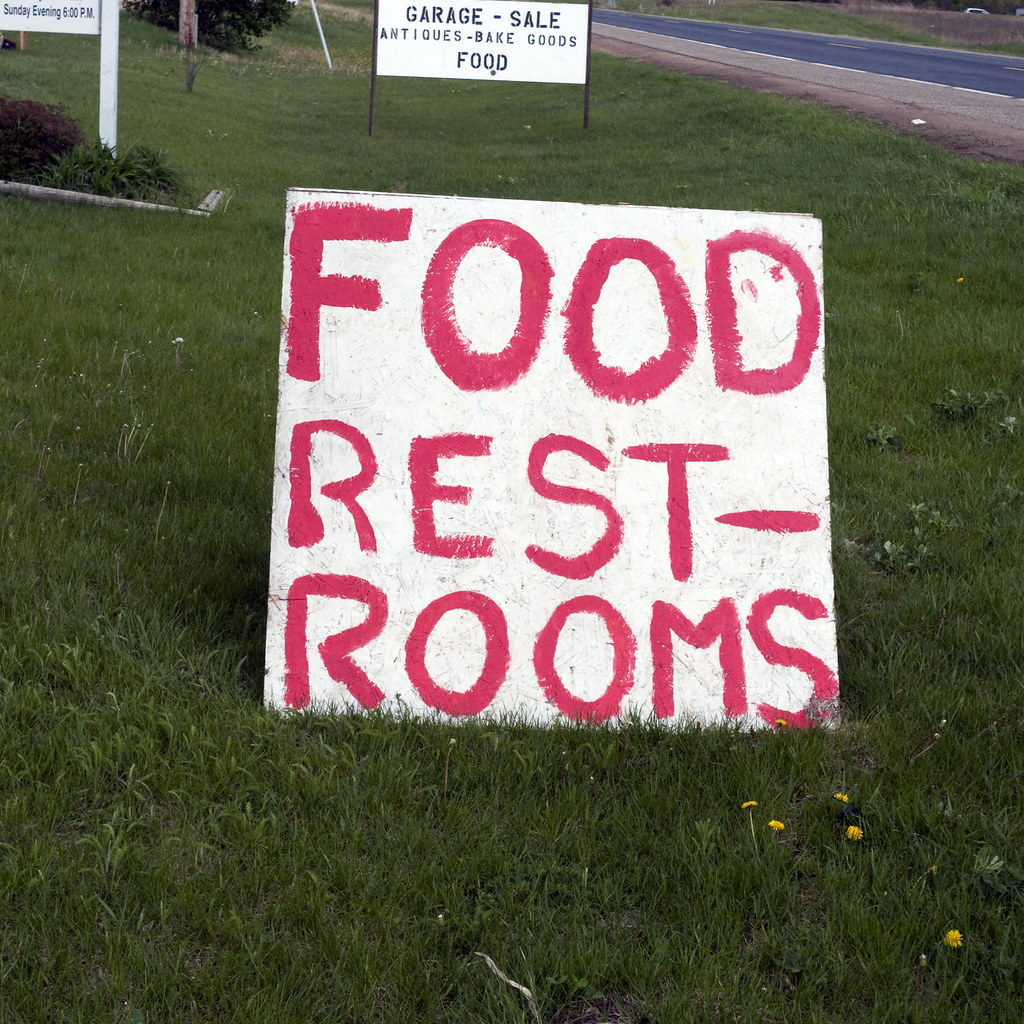The image showcases two signs, placed on a lush green lawn sprinkled with four blooming dandelions in the foreground. To the right of the scene, a road runs parallel to the signs' position. On the left, a prominent billboard advertises various services or products. The handmade sign in the forefront features a white background with large, bold, red letters reading "FOOD, RESTROOMS." Positioned behind this sign, another display appears crafted with stick-on letters, spelling out "GARAGE SALE, ANTIQUES - BAKED GOODS, FOOD." Notably, the word "baked goods" is repeated twice, likely for emphasis. A small twig is visible on the ground in front of the signs, adding a touch of natural detail to the setting.